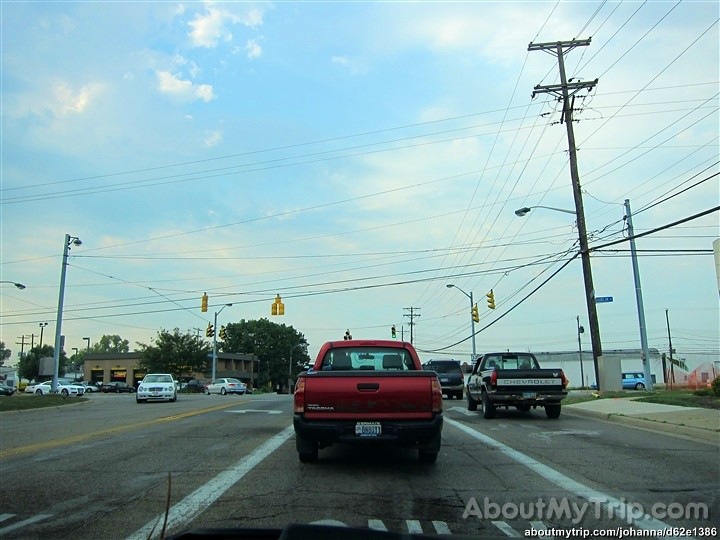The image captures a color photograph of a busy, muted intersection, viewed from an unspecified vehicle in traffic. Directly ahead is a red pickup truck, clearly visible with its tailgate, back window, and license plate. To the right, a black Chevrolet pickup sits in the right-hand turn lane. An oncoming white car approaches in the opposite lane. The scene unfolds at a four-way intersection, governed by seven traffic signals. Overhead, utility poles with crisscrossing power lines stretch across the blue sky dotted with wispy clouds.

To the right and left of the red truck, white lanes mark the grey road, while a central yellow line navigates the flow of traffic. The intersection features remnants of greyish buildings and scattered trees, adding to the urban landscape. In the lower right-hand corner of the image, a watermark reads, "AboutMyTrip.com," with additional text, "AboutMyTrip.com Backslash Johanna Backsplash D62E1386," marking its origin. Some more vehicles, including distant white cars, blend into the scene, enhancing the portrait of a congested urban roadway.